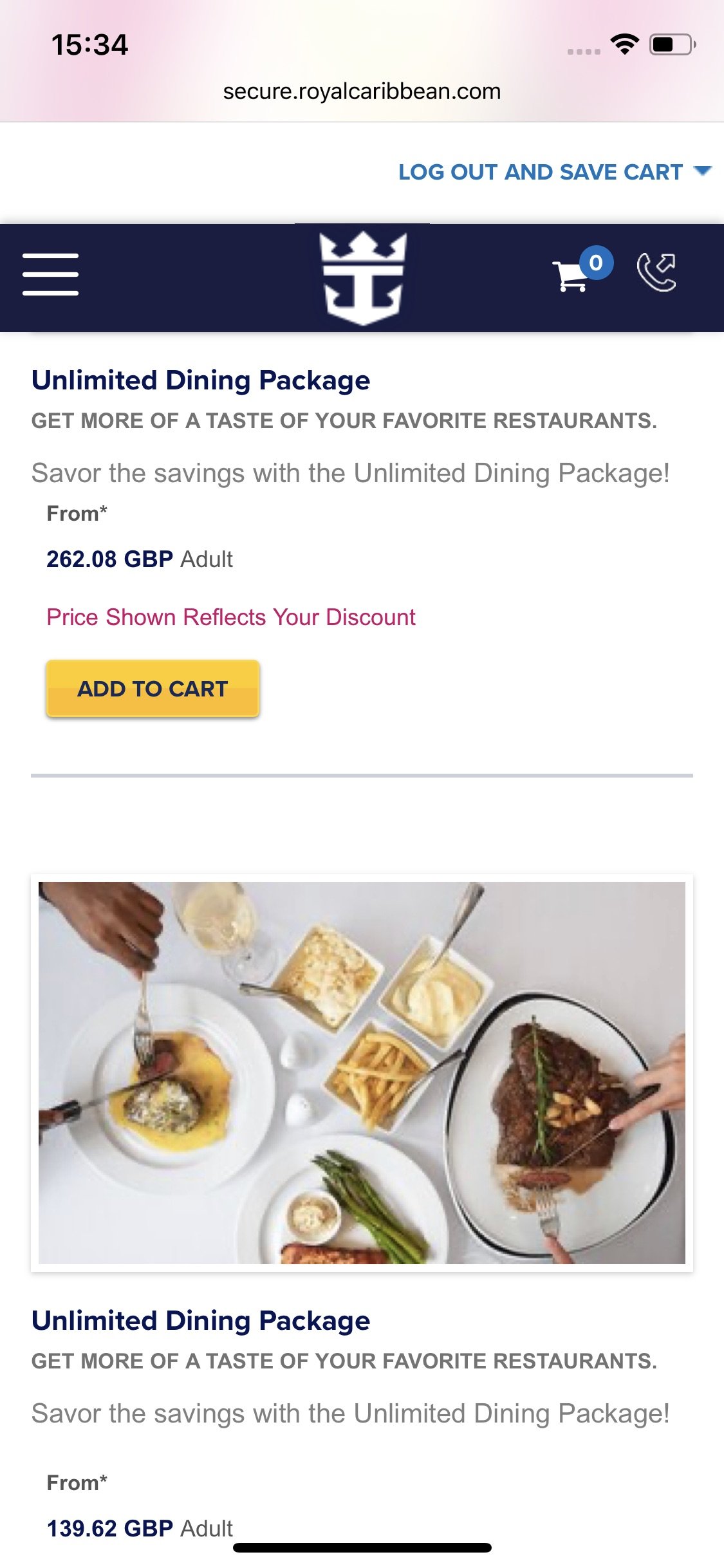The image portrays a detailed interface of a website, presumably for booking or browsing services related to "Roy Caribbean." The top section of the screen displays a rectangular banner with a gradient background transitioning through very light pink to beige and back to light pink. On the left, the time is shown as "15:34." In the center, the URL "secure.roycaribbean.com" is prominently displayed.

To the right, a series of icons include four gray boxes, a fully black Wi-Fi signal icon, and a battery indicator, which appears to be more than 50% charged. This area also features a logout option in bold, uppercase blue letters against a white background: the text reads "LOG OUT AND SAFEGUARD," followed by a downward-pointing triangle in the same color scheme.

Below this, there is a navy blue section with three white lines on the left. This section also includes a white icon of an ink with a crown, a shopping cart with a blue circle containing a white "0," and an icon of a phone with an upwards-diagonally pointing arrow.

Further down, a promotional area is set against a white background. The first line, written in blue text, reads "Unlimited Dining Package." Below this, in gray text, it encourages visitors to "get more of a taste of your favorite restaurant and savor the savings with the unlimited dining package." Next to an asterisk, the price "262.00 GBP" is displayed in blue, followed by the word "adult" in gray. A red note indicates that "the price shown reflects your discount." 

A yellow 'Add to Cart' button is prominently displayed in blue text just below these details. This section is divided by a thin gray line, and the bottom part of the image showcases various food items, including fries, asparagus, and steak, possibly illustrating the dining options available.

Overall, the image combines functional website elements with enticing visual details of dining options, aiming to engage the user and encourage them to avail themselves of the services offered.